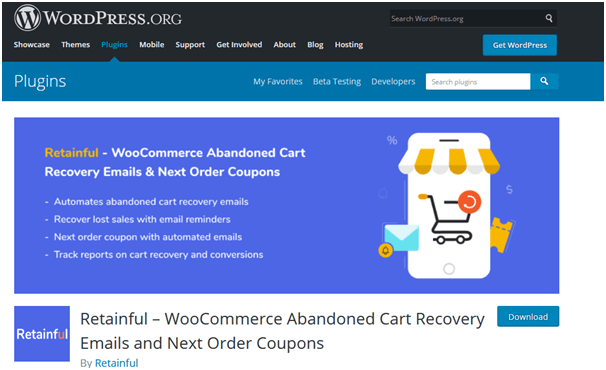In this image, the top portion features a large black box with a prominent "W" inside a gray circle, which is encircled by an additional gray ring. This icon represents WordPress.org. Adjacent to it, various menu options are listed including "Showcase," "Themes," and "Plugins," which are highlighted in blue with a small upward-pointing arrow. Other menu items such as "Mobile Support," "Get Involved," "About," "Blog," and "Hosting" are also displayed. On the top-right corner, there is a search button for easy navigation. Below this, a blue button labeled "Get WordPress" is prominently displayed.

Further down, a blue box contains options like "Plugins," "My Favorites," "Beta Testing," and "Developers," along with another search bar for plugin searches. The main background of this section is white, contrasting sharply with another blue box that showcases "Retainful" in orange text. This section specifies that it is related to "WooCommerce Abandoned Cart Recovery Emails and Next Order Coupons."

A detailed list follows, featuring bullet points:
- Automates abandoned cart recovery emails
- Recover lost sales with email reminders
- Offer next order coupons through automated emails
- Track reports on cart recovery and conversions

On the right side, there is a small white box with symbols including a percentage sign on the left and a dollar sign on the right. An icon resembling a telephone booth with an orange and white striped awning sits below these symbols. The booth contains a grocery cart and a red circle featuring a half-circle inside, as well as a blue envelope adorned with a yellow circle and a bell icon. One side of the icon looks like a yellow ticket and the other side features a small circle at the bottom.

The white background extends to the lower part where a small blue box lists "Retainful" in white text, except for the "U," which is orange. The text reads: "Retainful WooCommerce Abandoned Cart Recovery Emails and Next Order Coupons by Retainful," accompanied by a blue download button.